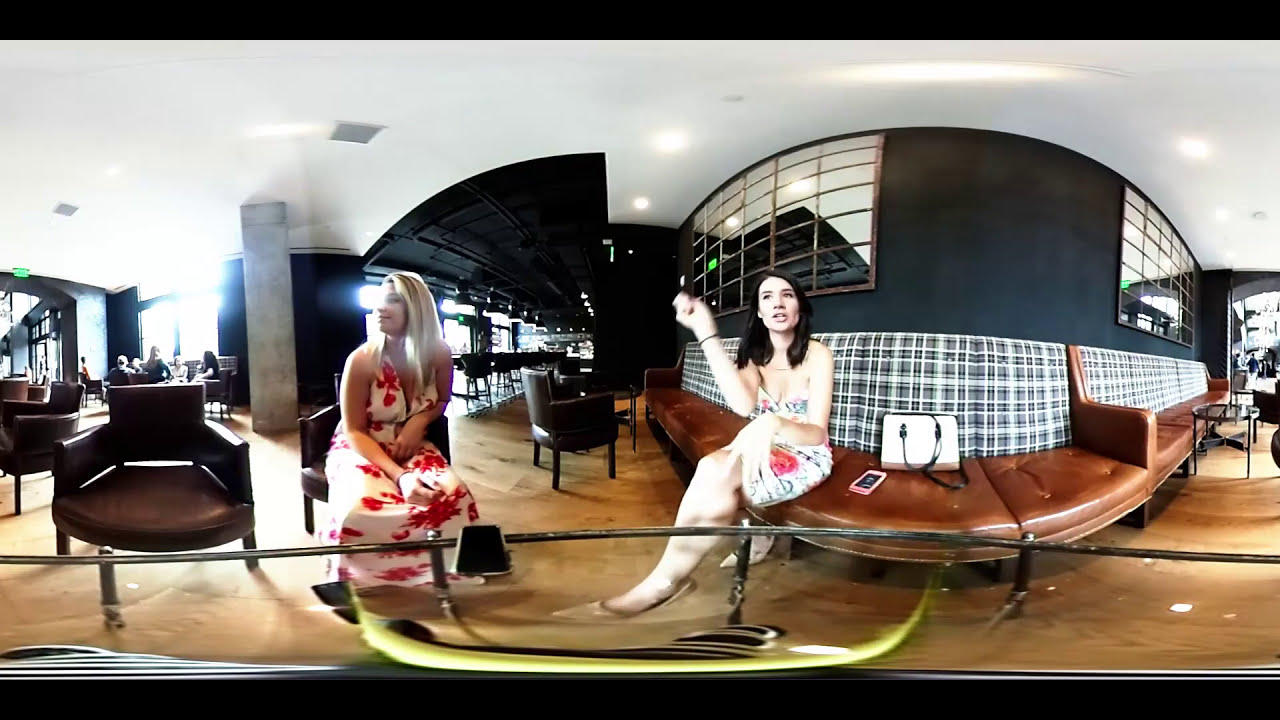In a slightly distorted fisheye cell phone image, two young women in their late 20s are seen inside what appears to be a hotel lobby or a restaurant/office meeting area. The woman on the right is seated on a brown leather couch adorned with a checkered blue and white cushion background. She has long dark hair that frames her face and shoulders, light skin, and wears a black watch band on her right wrist. Her white purse and phone rest on the couch beside her. She appears to be mid-conversation, looking almost directly at the camera with a slight blur indicating movement. 

On the left, the second woman sits in a chair with her hands resting on her lap. She has long blonde hair flowing down to her chest and wears a distinctive sleeveless white dress with red splotches, resembling red flowers. She has a nonchalant expression and gazes off to the left, away from the camera. Visible on a glass table in front of her is her phone. In the background, additional people are grouped together, adding to the lively atmosphere of the setting.